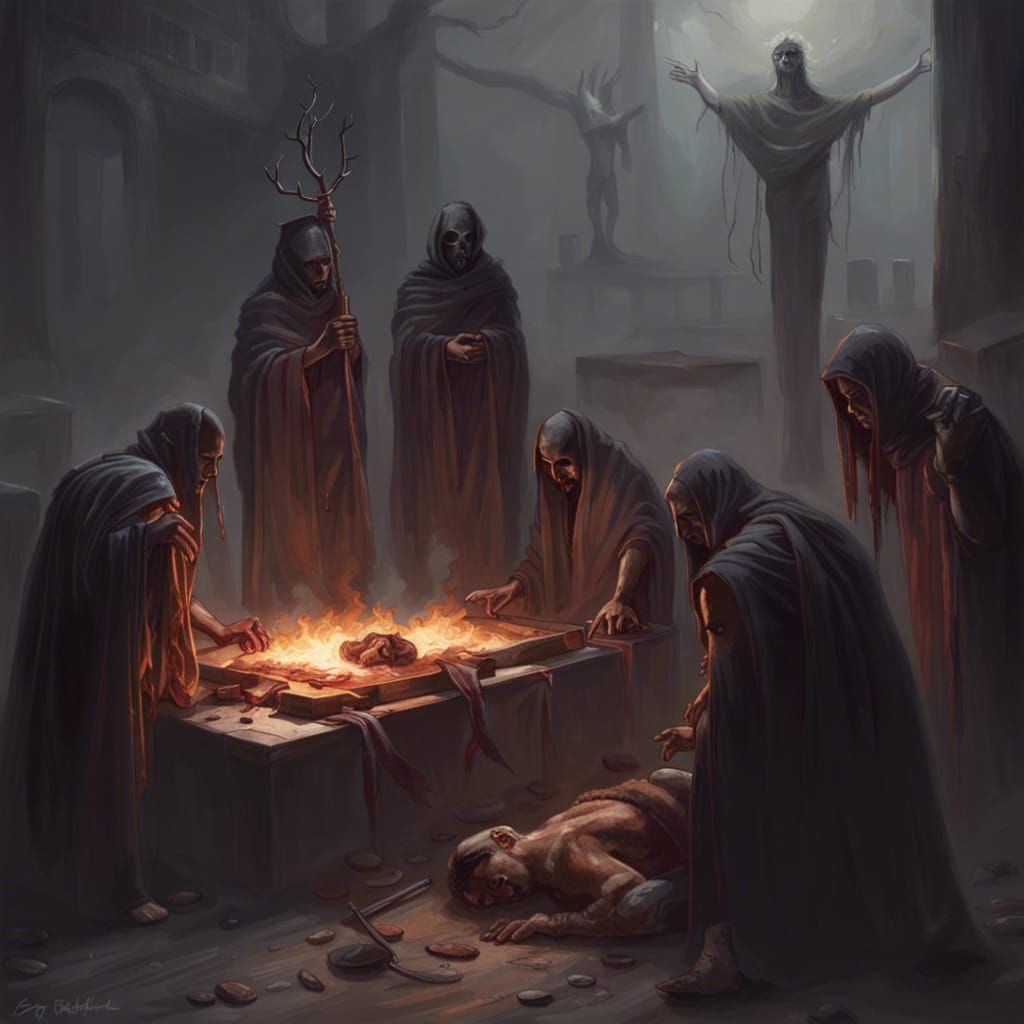The painting depicts a dark, gothic scene set within a dungeon-like environment with tall, gray, concrete walls, shrouded in smoke and dim, eerie light. At the center, there is a large rectangular stone table or altar with a fire burning in its middle, strips of clothing draped over its sides. Surrounding the altar are ghoulish figures in black robes, their faces skeletal with hollowed eyes, invoking an atmosphere of dread. One of the central witches or ghouls wields a golden staff topped with antler-like branches. 

In front of the altar lies a deceased man, his upper body exposed and face down on the cold, stone floor. Two robed figures loom over him, possibly engaged in some dark ritual. The background is populated with unsettling statues: one resembling a person with outstretched arms shrouded in a long dress and shawl, another featuring a human body from the neck or chest down with a mask of a wolf or similar creature placed on top.

The overall ambience is one of dread and horror, with the scene potentially taking place in a cursed graveyard or ruin, adding to the macabre feel.